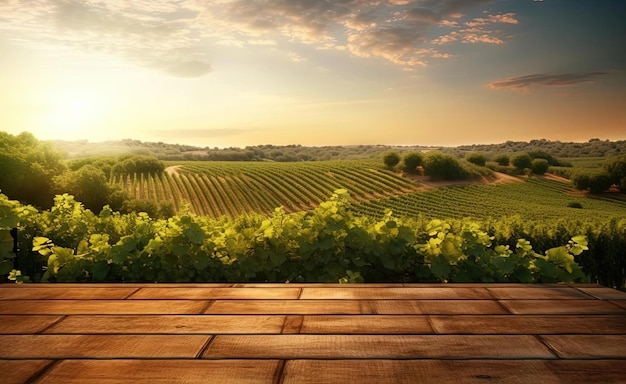In this detailed scene, the viewer's perspective appears to be from a wooden deck or platform in the foreground, characterized by brown, perfectly shaped planks. Immediately beyond the deck lies a line of leafy, light green foliage. Stretching out past this greenery is an expansive, open field with meticulously straight rows of planted crops, although the specific type of crop remains unidentifiable. To the right side of the field, a few small trees are interspersed among the crops. This vibrant field is set against a backdrop of a densely forested area, adding depth to the landscape.

Above the fields, the sky presents a picturesque transition from sunset's warm hues to cooler tones. The sun, shining brightly from the left, illuminates the scene beneath a scattering of white clouds that stretch across the sky, adding texture and contrast to the vivid mixture of oranges and blues. The horizon glows orange from the setting sun, fading upward into the deepening blue of the evening sky.

The entire scene exudes tranquility and the promise of growth, with the neatly planted rows suggesting a land well-tended and cherished. The photograph captures the balance between human cultivation and natural beauty, evoking a sense of peaceful solitude and connection to the rural landscape.